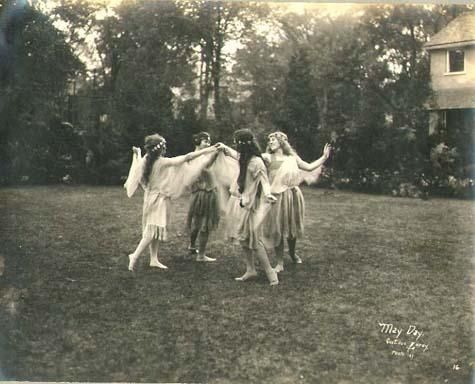This square, black-and-white photograph exudes a nostalgic charm, showcasing its age with visible light leaks and chromatic aberrations indicative of analog photography. Set against a backdrop of lush trees and bushes, and partially obscured in the upper right corner by the side of a two-story house, the scene centers on four young women. Dressed in fringed, flowy dresses characteristic of the early to mid-1960s and adorned with flowers and headbands in their long hair, the girls stand barefoot on a freshly mowed lawn. They hold hands in a circle, appearing to dance joyfully, their expressions reflecting the merriment of the moment. The text "May Day" is faintly visible at the bottom right, accompanied by three other nearly illegible lines, suggesting a possible celebration or event, further evoking a sense of bygone times.